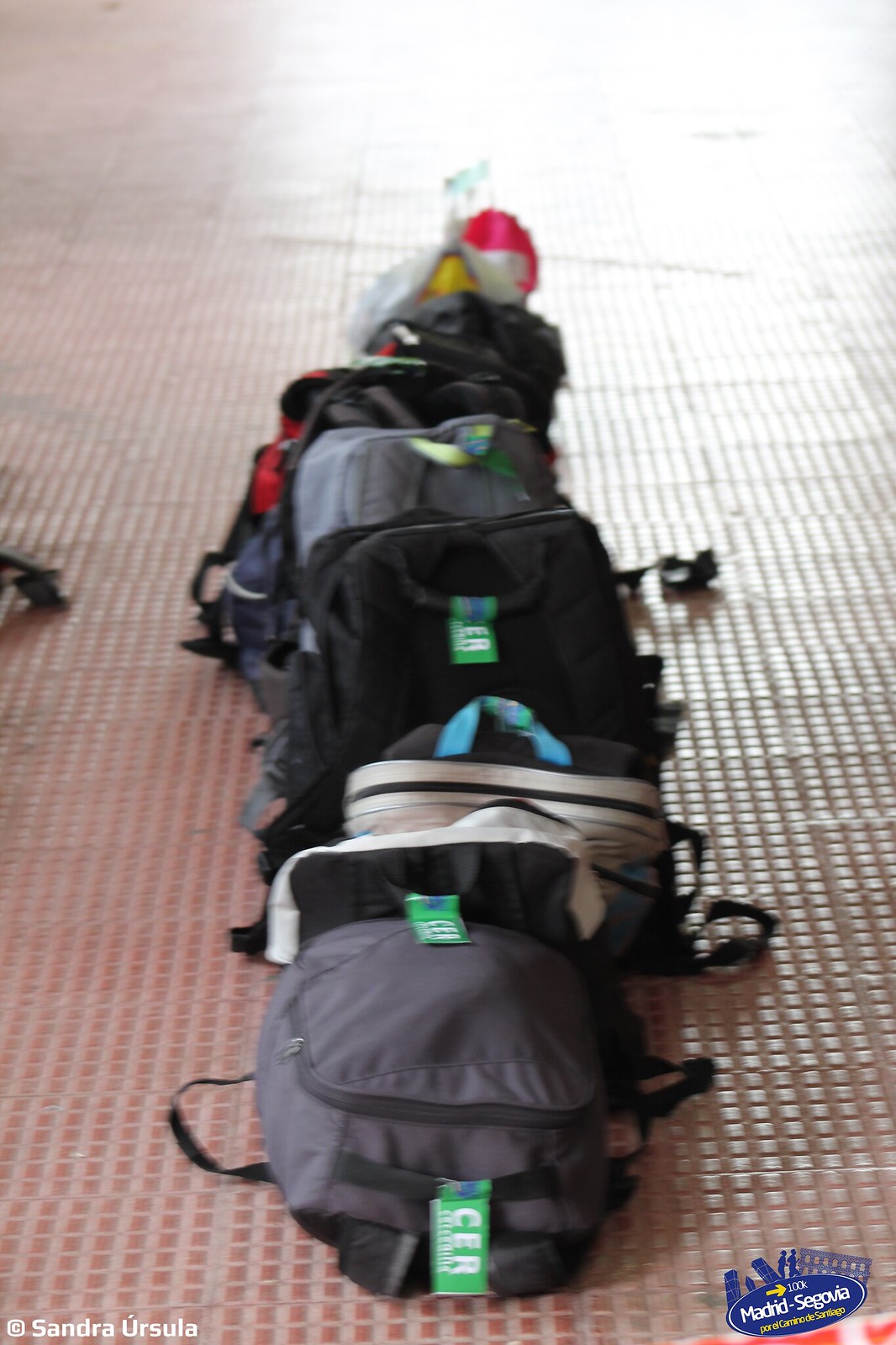The image captures a slightly out-of-focus row of backpacks arranged vertically, receding into the distance. Most of the bags are gray, but there are splashes of color with one or two hints of red and a possible yellow bag further back. One particular bag is white with a black zipper, while another has a black strap area. The bags appear to be either standing up or leaning against each other, maintaining the line's overall shape. The backpacks rest on a rubbery checkered mat that's pale pink with darker pink squares interspersed in a regular pattern. Bright, possibly natural sunlight glares from the top middle right, creating a bright white haze that obscures some details. Several bags have green tags with the letters "C.E.R." visible. 

In the lower right corner, there is a blurred logo with a yellow arrow and small unreadable white text, beneath which it says "Madrid, Segovia," surrounded by an oval shape decorated with symbols of buildings and people. In the bottom left corner, the image bears the white text "copyright Sandra Úrsula," with an accent on the first "U". Below this text, there are blurred red and white elements in the picture. This photograph likely depicts a group of travelers' backpacks, suggesting a journey from Madrid to Segovia.